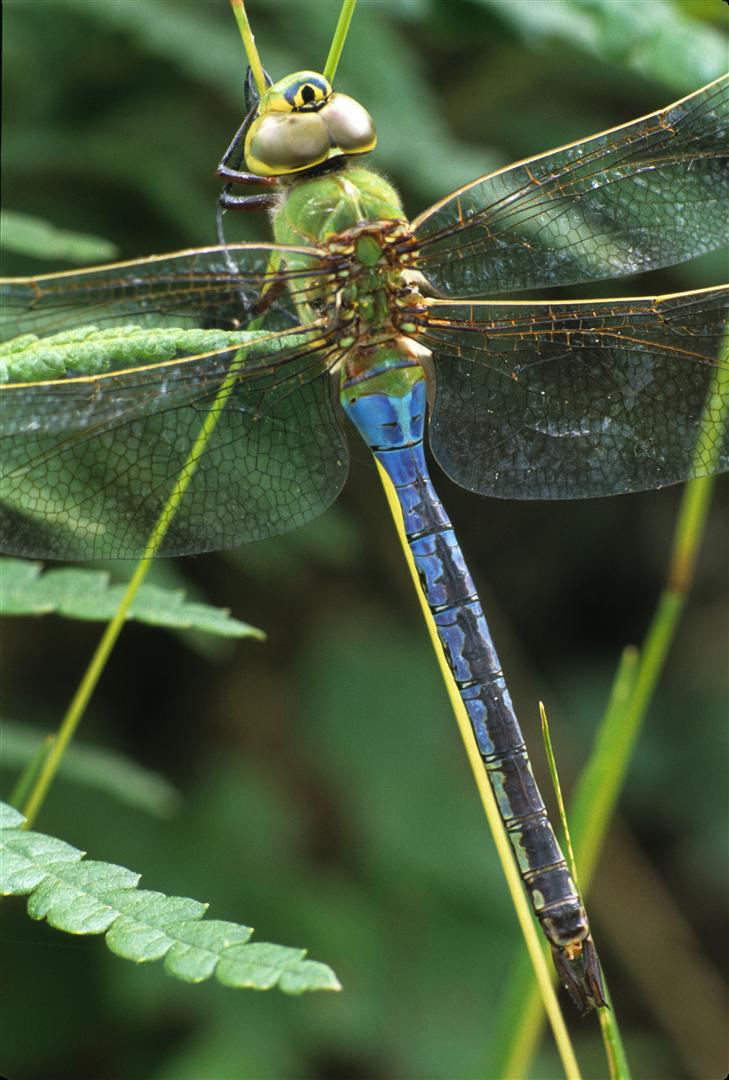This high-resolution, top-down photograph captures an intricately detailed dragonfly perched among green and light green leaves. The dragonfly's body features a striking brilliant blue tail, contrasting with its predominantly green thorax to which four clear wings with a delicate black lace pattern are attached. The front edges of these wings are accented with a subtle yellow stripe. The head of the dragonfly presents a fascinating visual illusion, resembling a cyclopean face with one large central black eye surrounded by yellow and blue rings, complemented by what appear to be white, puffed-out cheeks. Additionally, this natural yet almost surreal visage is further adorned with green antennae extending upwards. The image also highlights three of the dragonfly's six legs, meticulously detailed against a blurred leafy background that accentuates the focus on the intricate structure and vibrant colors of the insect itself, showcasing the complexity and beauty of the natural world.